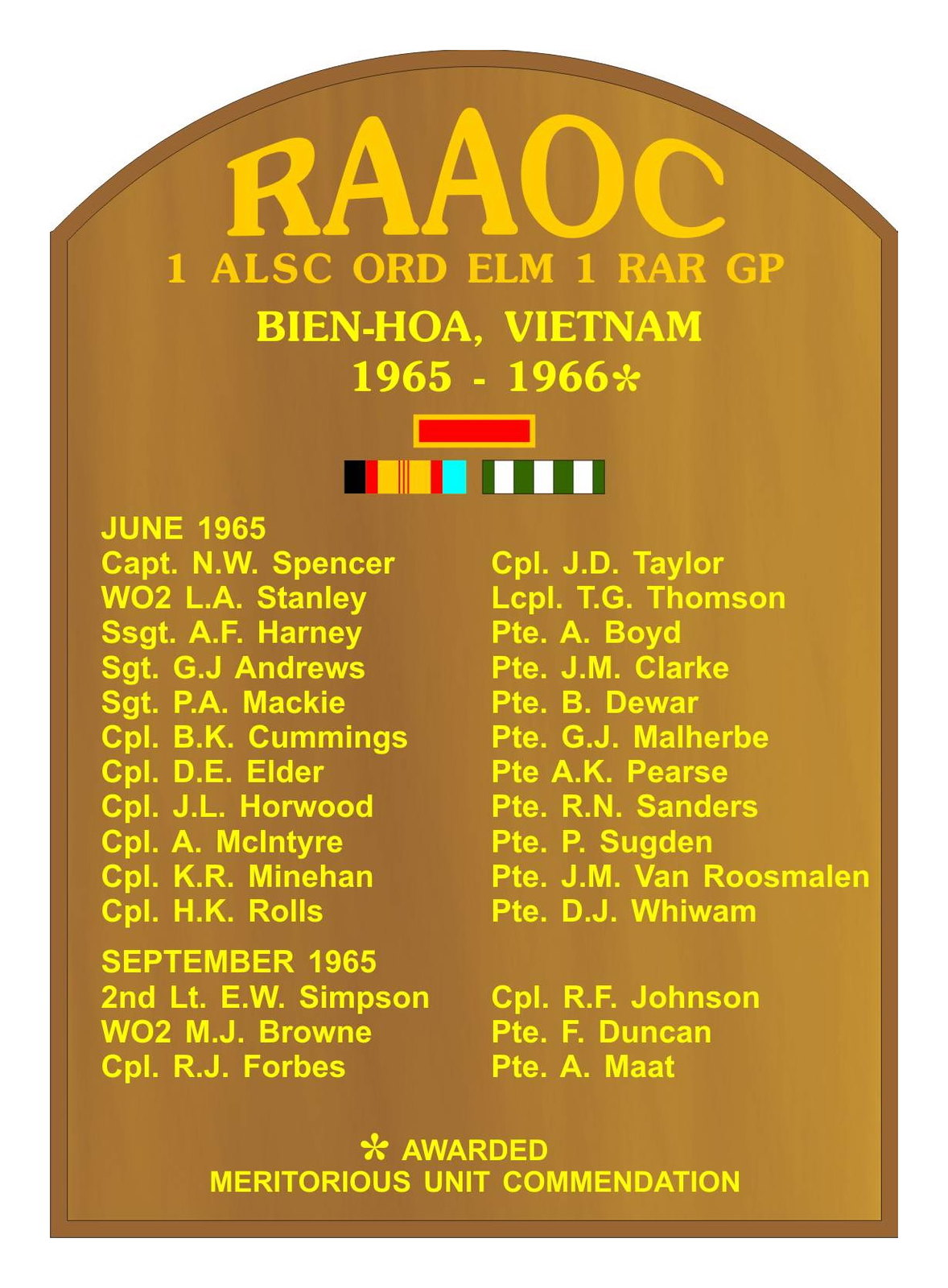The image portrays a digitally synthesized headstone-shaped plaque, rendered in a textured dark brown wood color. At the top, prominently centered, is the acronym "R-A-A-O-C" written in large yellow capital letters. Below this, in smaller yellow font, is "1-A-L-S-C ORD ELM 1-R-A-R-G-P." The inscription "Bien Hoa, Vietnam" follows in brighter yellow, accompanied by the dates "1965 to 1966" with a star beside it. Beneath this, a red rectangular bar with an orange outline is centered, followed by two military rank bars—one in black, red, orange, and blue, and the other in white and green.

The lower portion of the plaque features two columns of names, categorized by the months "June 1965" and "September 1965." These names are written in both red and yellow, denoting the rank, first initials, and last names of individuals. Positioned at the bottom of the image is a yellow star next to the inscription "awarded Meritorious Unit Commendation." The plaque is centered within the digital canvas, serving as a remembrance for those who served in the Vietnam War.